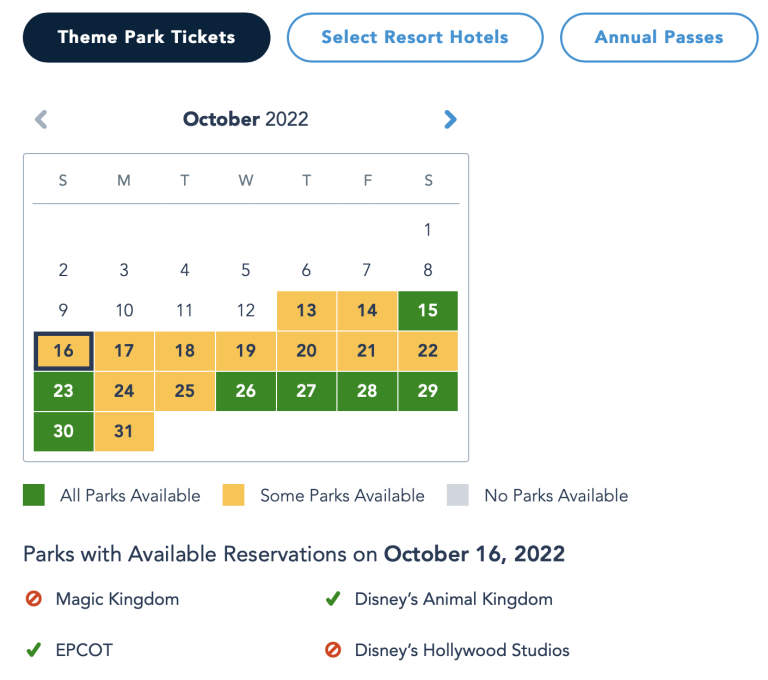This image depicts a section of a booking webpage. At the top of the page, there are three selection bubbles. The first bubble, labeled "Theme Park Tickets," is highlighted in black, indicating it is currently selected. To the right, the next two bubbles, labeled "Select Resort Hotels" and "Annual Passes," are in blue and white, suggesting they are not currently selected.

Below these bubbles, on the left side, the text "October 2022" is displayed with a calendar for that month beneath it. The calendar shows the dates from the 1st to the 12th in a standard, unhighlighted format, while the dates from the 13th to the 31st are highlighted with varying colors. 

Most of the highlighted dates are in yellow, indicating that "some parks are available." However, specific dates—namely the 15th, 23rd, 26th, 27th, 28th, 29th, and 30th—are highlighted in green, which denotes that "all parks are available." Additionally, a color legend at the bottom of the calendar clarifies that gray signifies "no parks available." On October 16th, it is noted that Disney's Animal Kingdom and Epcot have reservations available.